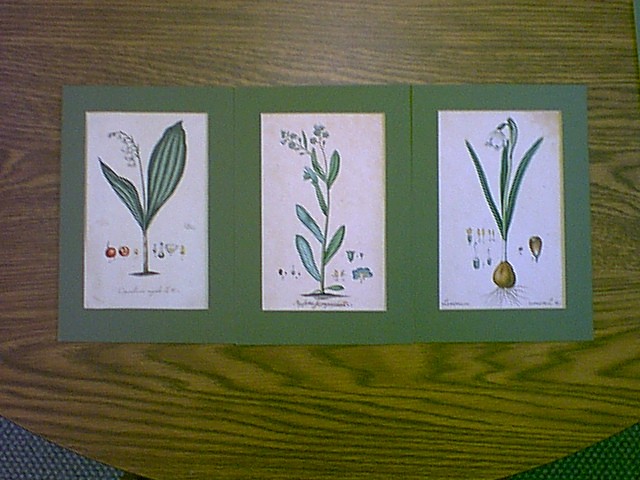This image features a set of three detailed botanical illustrations, each matted with green cardstock and arranged side-by-side, touching edges. The illustrations are presented on a blue-brown wooden table, creating a framed display with a clean white background. 

The first illustration on the left depicts a plant with two prominent, large green leaves adorned with white veining, accompanied by small white blossoms and various fruits. Beneath this illustration, there are some symbols or text, though they are not legible.

The middle image showcases a plant characterized by six smaller blue-green leaves arranged along a central stalk, topped with purplish flowers. This illustration also includes illegible characters below the drawing.

The third illustration on the right features a plant resembling a bulb, possibly an onion, at its base with roots extending downward. It has long, slender leaves growing upward and a delicate white blossom. Below this image are also characters or symbols that cannot be clearly read.

Overall, the meticulous botanical drawings create a vivid display of plant life, framed together in an aesthetically pleasing arrangement.